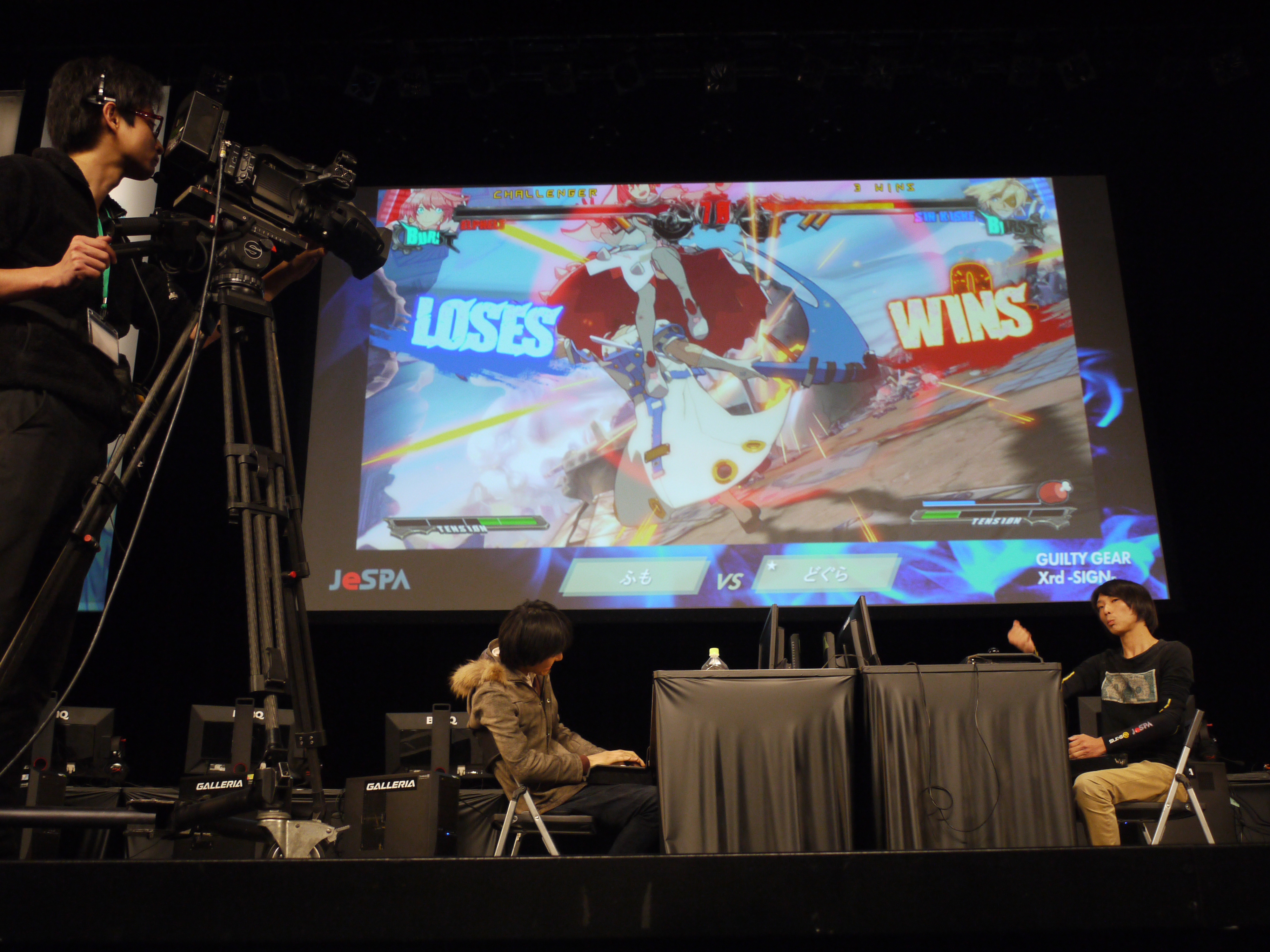In the photograph, the setting is a stage with a predominantly black background and a large screen displaying an anime-themed video game. The screen prominently features the words "Loses" in blue on the left and "Wins" in white on the right. The game visuals show two women, one airborne with visible legs, seemingly attacking another woman with red hair in a white dress. On the stage, there are two tables draped in black tablecloths. To the left, an Asian man sits with a laptop, wearing a brown jacket and black pants. To the right, another Asian man in a black long-sleeve shirt adorned with an emblem and tan pants is also seated. Between them, a person in glasses with short black hair, dressed in a black shirt and black pants, operates a large camera on a tripod-like stand, aiming it at the stage. This appears to be an event, possibly a comic con, where the individuals on stage are engaging with the game projected on the large screen behind them. The black backdrop enhances the vivid colors and dynamic visuals on the screen, heightening the focus on the competitive gaming scene being captured.